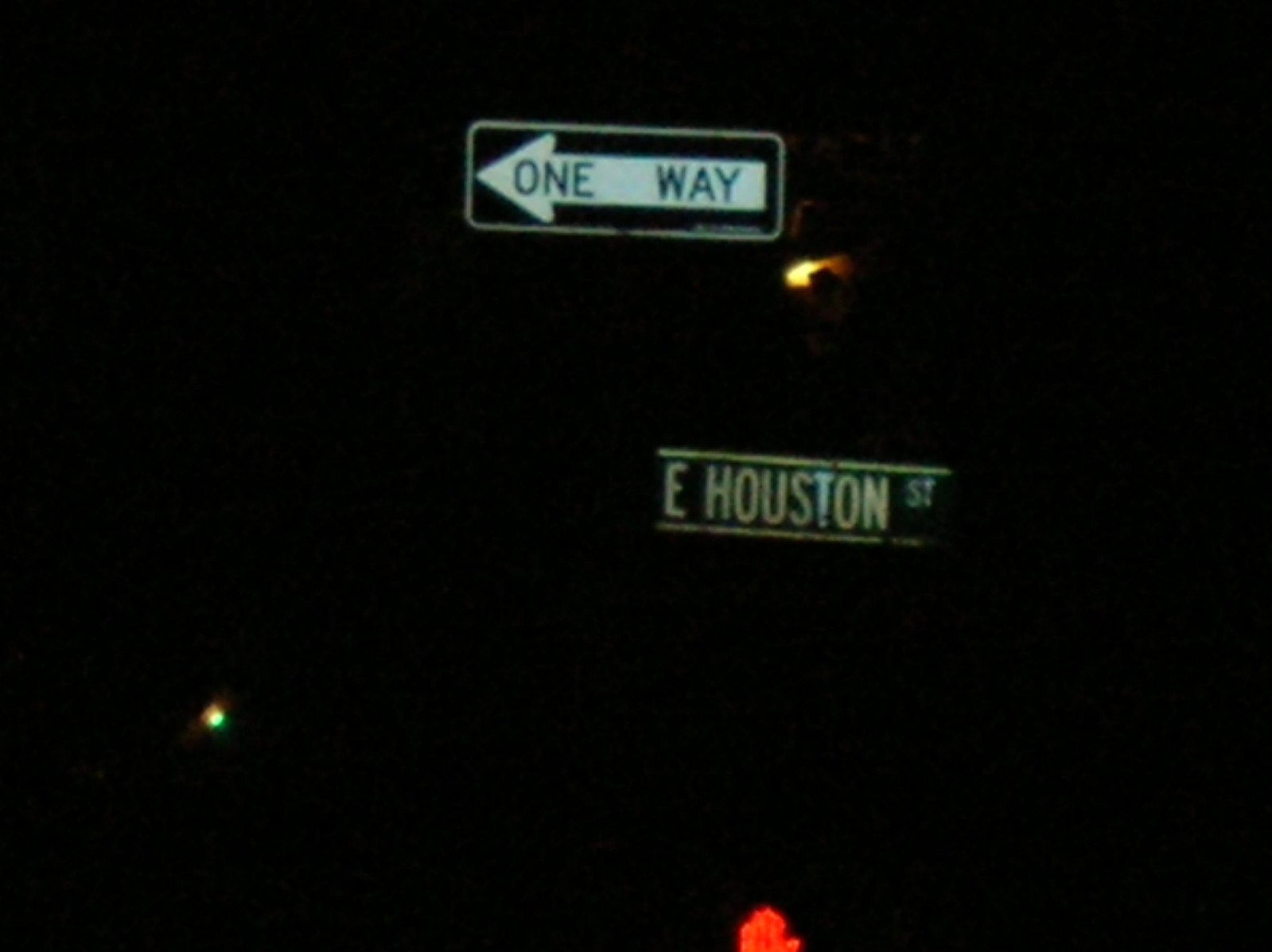This photograph, although dark and slightly blurry, captures an intricate nighttime street scene. The background is predominantly black, contributing to the dim atmosphere. Centered at the top is the faint outline of a rectangular street sign with a white rim. The sign features a white arrow pointing to the left, with the words "One Way" inscribed in black on the arrow. Below the sign, to the bottom right, an orange-yellow curved area indicative of a streetlight casts a subtle glow. Below this and slightly to the right, another street sign is visible, displaying the text "E. Houston Street" against a black background, framed by white lines at the top and bottom. Towards the left edge, nearer to the bottom of the photograph, there is a small, blurred white light. Additionally, off-center at the very bottom right, a larger, semi-circular blurred light with a small protrusion on the right side adds an abstract touch to the composition.